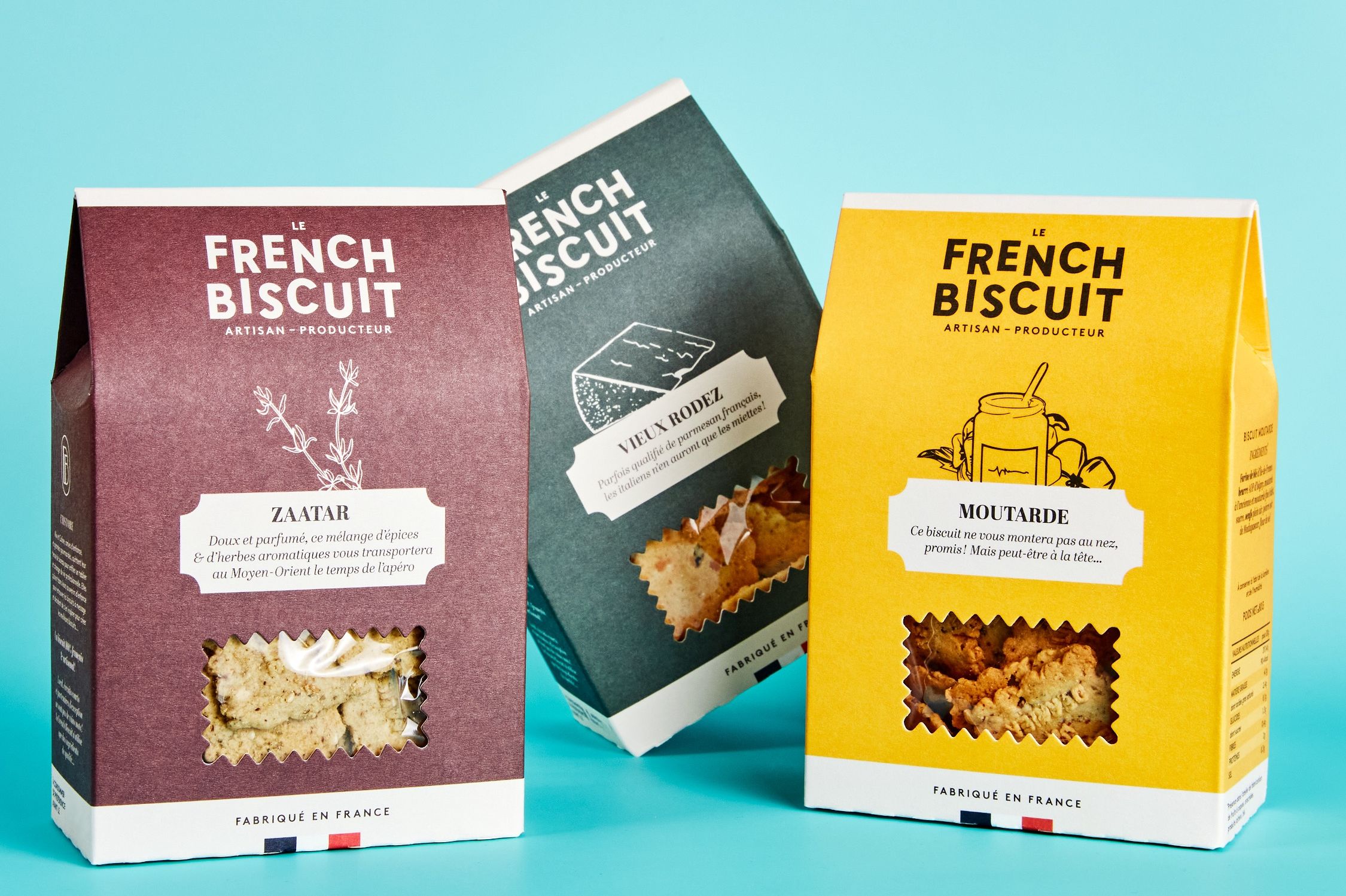This advertisement features three different flavors of Le French Biscuit Artisan Producteur's specialty crackers, set against a pale blue background. The crackers are displayed in three distinct, partially transparent bags with identical design elements but different colors. The leftmost bag is burgundy and contains za'atar-flavored crackers, depicted with a line drawing of herbs or seasoning. The middle bag, green in color, showcases Vieux Rodet crackers symbolized by a cheese block illustration. The rightmost bag is bright yellow, containing moutard (mustard) crackers, represented with a jar of mustard and spoon graphic. Each bag has white creased tops and bottoms with a black and red square denoting "Fabrique en France" – black on the left and red on the right. Nutritional information appears visible on the side of the yellow bag, adhering to typical labeling standards.